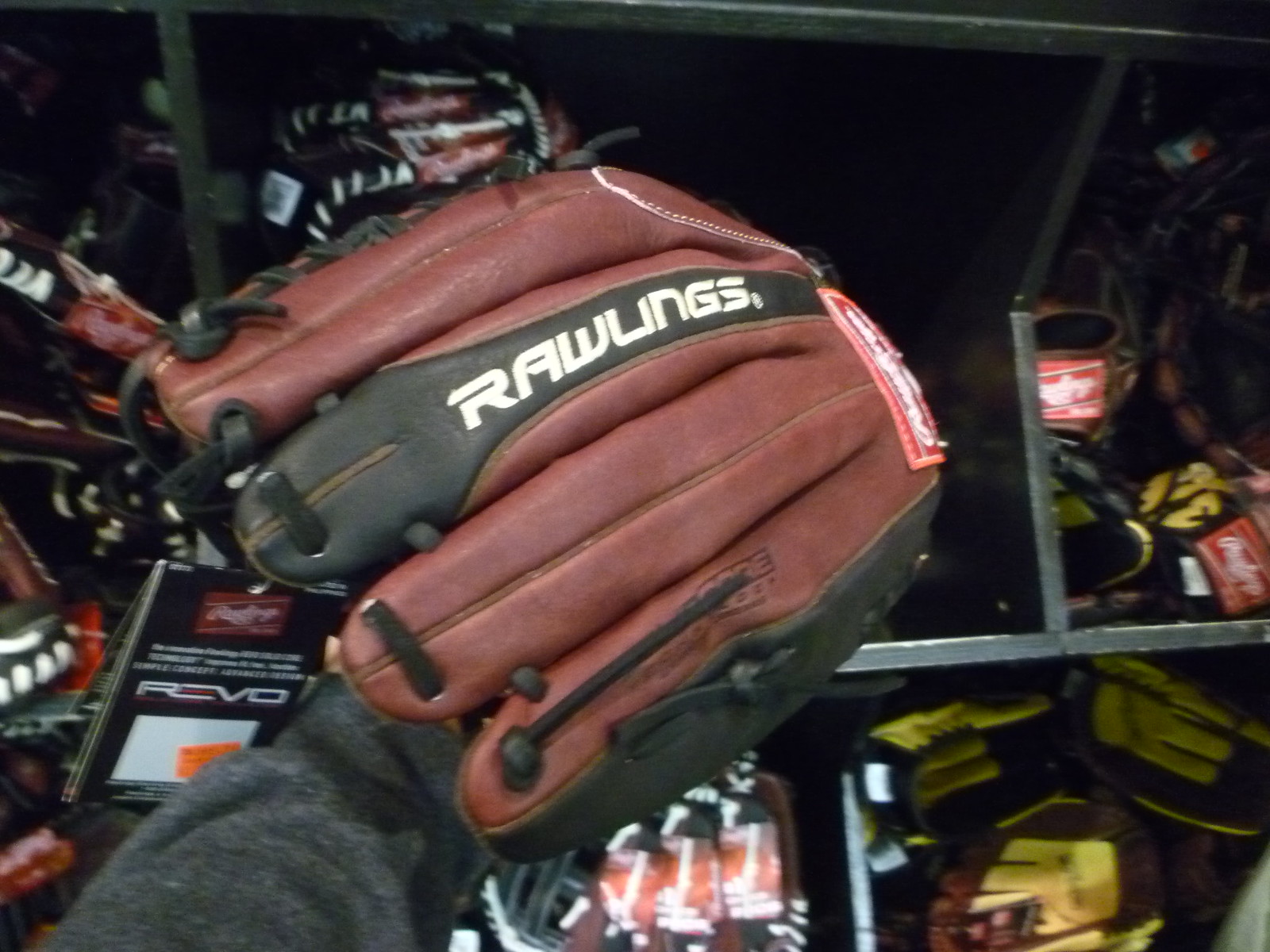The close-up image captures a Rawlings baseball glove prominently displayed in the center. The brown leather catcher's mitt is detailed with black lacing and a significant black leather piece along the fingers. The "Rawlings" brand is clearly stamped in white on this black strip, running along the middle finger of the glove. Extending from the bottom left of the image is an arm in a textured gray long-sleeve sweater, reaching towards and holding the glove in such a way that the hand is obscured. Surrounding the main glove, the background reveals shelves filled with various baseball supplies, including other gloves and possibly leather work gloves to the right. A red patch is visible near the top of the main glove, while below the sweatered arm, a "Revo" sign is faintly discernible. The image provides a detailed and contextual view of the glove within a store setting, showcasing its brand, design, and surrounding merchandise.